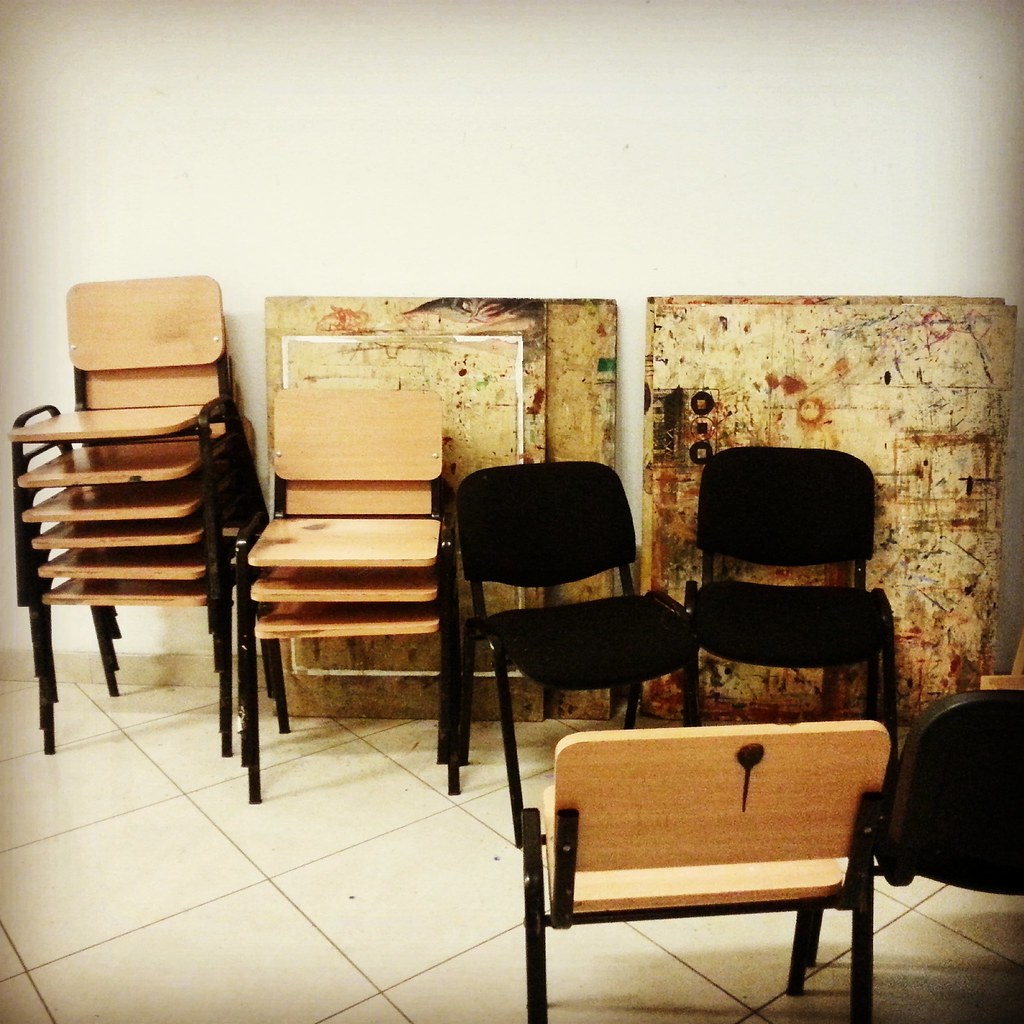In the color photograph, several stacks of chairs and individual chairs are arranged on a large tiled floor with light yellow tiles and dark grout lines. To the left, stacks of chairs with golden brown wooden seats and backs, supported by black metal legs, form rows. One stack has four chairs, and another has three chairs, with an additional single chair positioned with its back toward the bottom right corner, displaying a dark brown blotch. Nearby, two wooden boards, approximately four feet by four feet, are propped against a white wall, covered in splatters of various paints and possibly ink, suggesting usage as art panels or old window frames. In front of these boards, and slightly off to the right, cushioned chairs with black fabric seats and backs, complemented by black metal legs, stand out. The setting, which resembles a multipurpose community center or art studio, features additional black fabric chairs, emphasizing its potential creative and functional versatility.